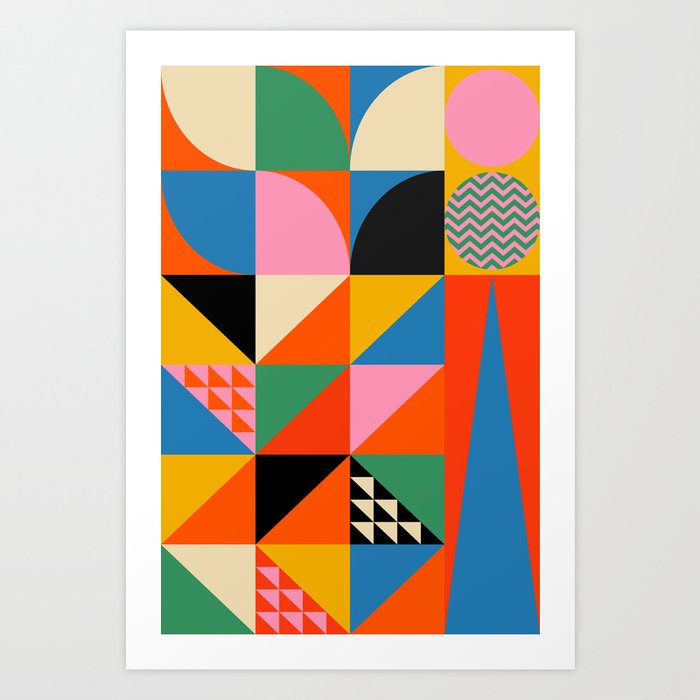The image is a photograph of an abstract painting or poster displayed vertically on a white wall. The artwork itself is framed with a white border and presents a modern, flat design characterized by a geometric and colorful array of shapes. Various squares, rectangles, and circles are filled with different patterns, including zigzags, half-moons, quarter circles, and triangles. A notable feature includes two circles within a rectangle, one of which is adorned with zigzag lines. The dominant colors in the painting are red, green, black, blue, yellow, pink, beige, and orange. Each shape is divided into sections with contrasting colors and patterns—a grand triangle on the right stands out with its blue hue juxtaposed against a reddish-orange background. The composition is a lively blend of color and form, lending to its distinctly modern and abstract style.